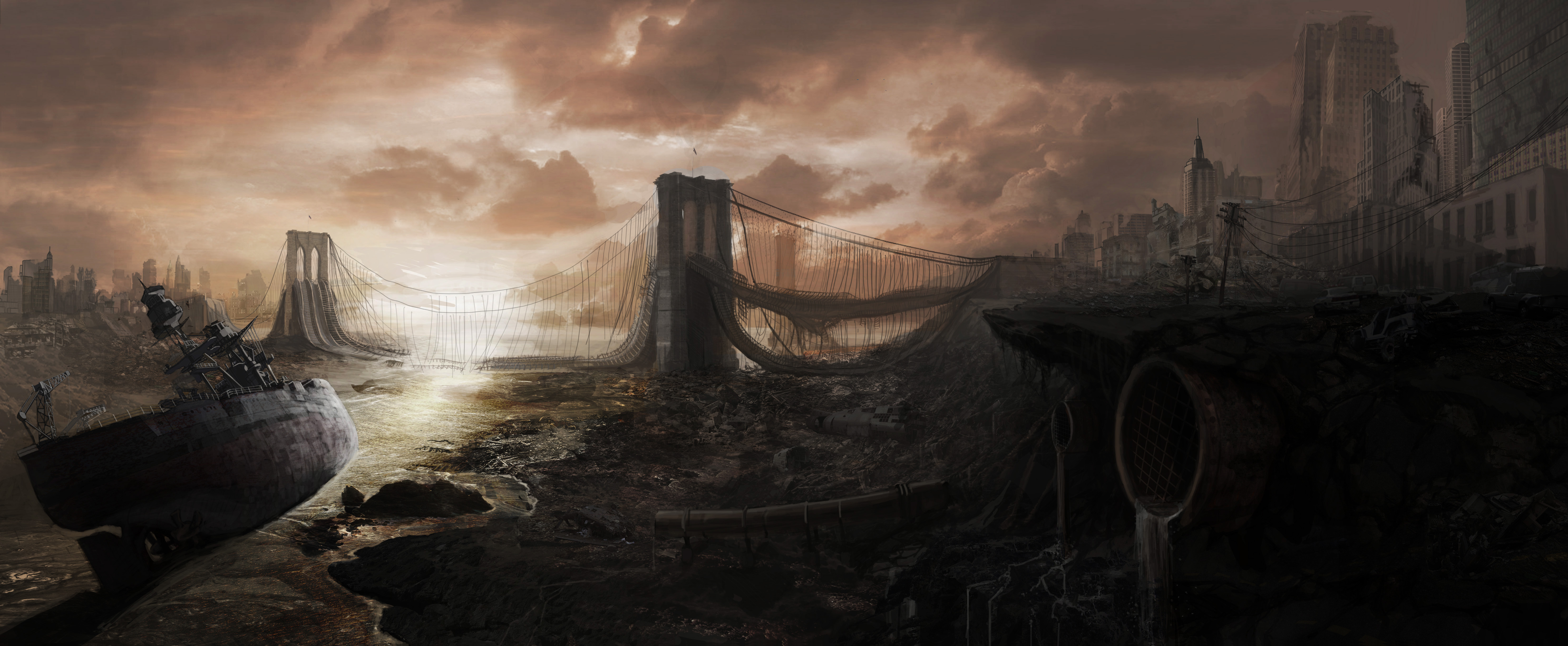The artwork presents a detailed, post-apocalyptic cityscape with an array of ruined structures and a haunting atmosphere. On the right side, a series of crumbling skyscrapers stands in stark decay, with telephone wires and poles in disrepair. A large drain pipe intermittently releases water into a dry, eroded riverbed. The centerpiece of the left side is the remains of a large suspension bridge, reminiscent of the Brooklyn Bridge, its support pillars and dangling wires hauntingly intact while the main span has collapsed into what once was a flowing river. The river is now a dried-out expanse of mud, littered with a military ship listing on its side, testament to a bygone era of devastation. In the distance, more skeletal buildings loom under an ominous sky tinged with an orangish tan hue. Patches of the gray clouds part to reveal faint rays of light, suggesting the presence of a hidden sun, subtly illuminating the scene in the upper middle portion of the image. The overall mood is one of somber desolation, capturing a world long fallen into ruin.